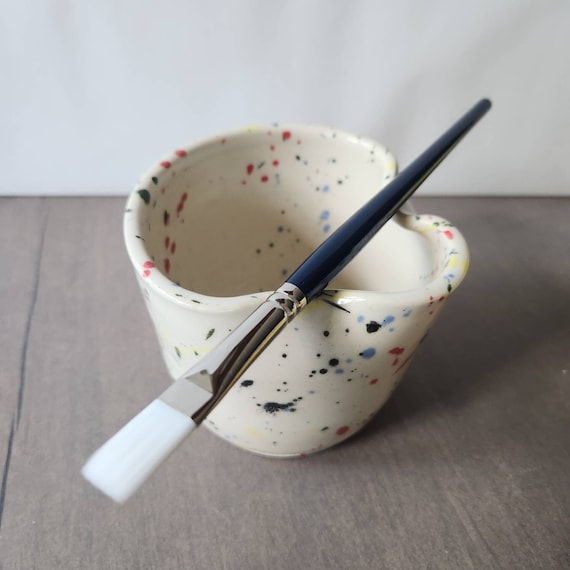The image showcases a close-up photograph of a unique white ceramic pot, which is speckled with various colors of paint—red, blue, black, and yellow. This small, lidless vessel, resembling a tulip shape and featuring an unusual fluted lip or pinched section on the right side, sits centrally on a tan wooden table. Across the unusual lip, a brand new paintbrush with pristine white bristles and a blue wooden handle is balanced diagonally. The brush's silver ferrule shines, holding the bristles firmly as they point towards the lower left corner of the frame. The background appears to be a white wall or backdrop, potentially resembling paper with a slight ripple effect, providing a clean, neutral contrast to the artistic tools. The entire scene gives the impression of readiness for an artistic endeavor, with the pristine condition of the paintbrush and the colorful, paint-splattered pot inviting creativity.